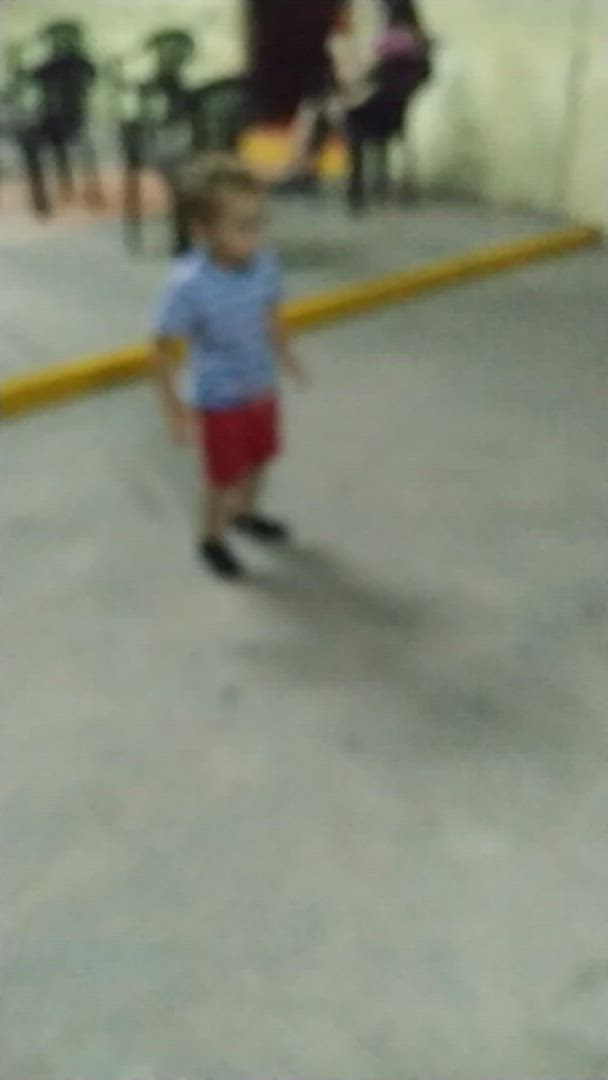In this out-of-focus and very blurry image, a young boy, approximately four years old, is captured mid-step. He is dressed in red shorts and black shoes, complemented by a short-sleeved shirt that seems to be a combination of white and blue. He strides forward with both hands slightly out to his sides, perhaps to maintain balance or in joyful motion. The boy walks on a gray concrete floor, and behind him, there is a yellow-painted curb-like step. The background features indistinct forms of people who are either standing or sitting, difficult to discern due to the image's lack of clarity. The scene is set against a backdrop of what appears to be a concrete wall, adding to the industrial feel of the environment.